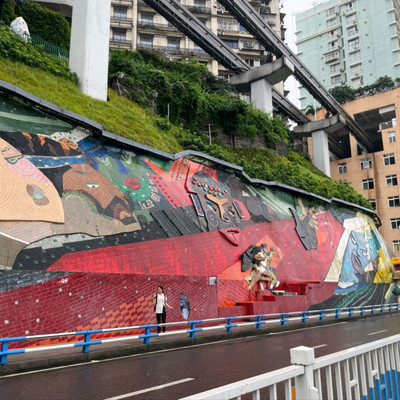The image captures a vibrant hillside mural predominantly featuring red and black hues with abstract faces. A black road marked with white stripes runs across the foreground, flanked by a blue and white railing that serves as a protective barrier for pedestrians. To the right of the mural, a person is seen walking, adding a sense of scale to the massive artwork. The mural itself appears almost three-dimensional, with various abstract figures and splashes of green embedded within its design. Above the mural, lush green grass and trees blanket the hillside, providing a striking contrast to the urban elements below. The top left portion reveals a railway and some light-colored buildings—orange, light brown, and light green—all interspersed with trees and white pillars, through which train tracks seem to weave in and out. Overall, the photo encapsulates an intricate blend of natural beauty, urban infrastructure, and artistic expression.